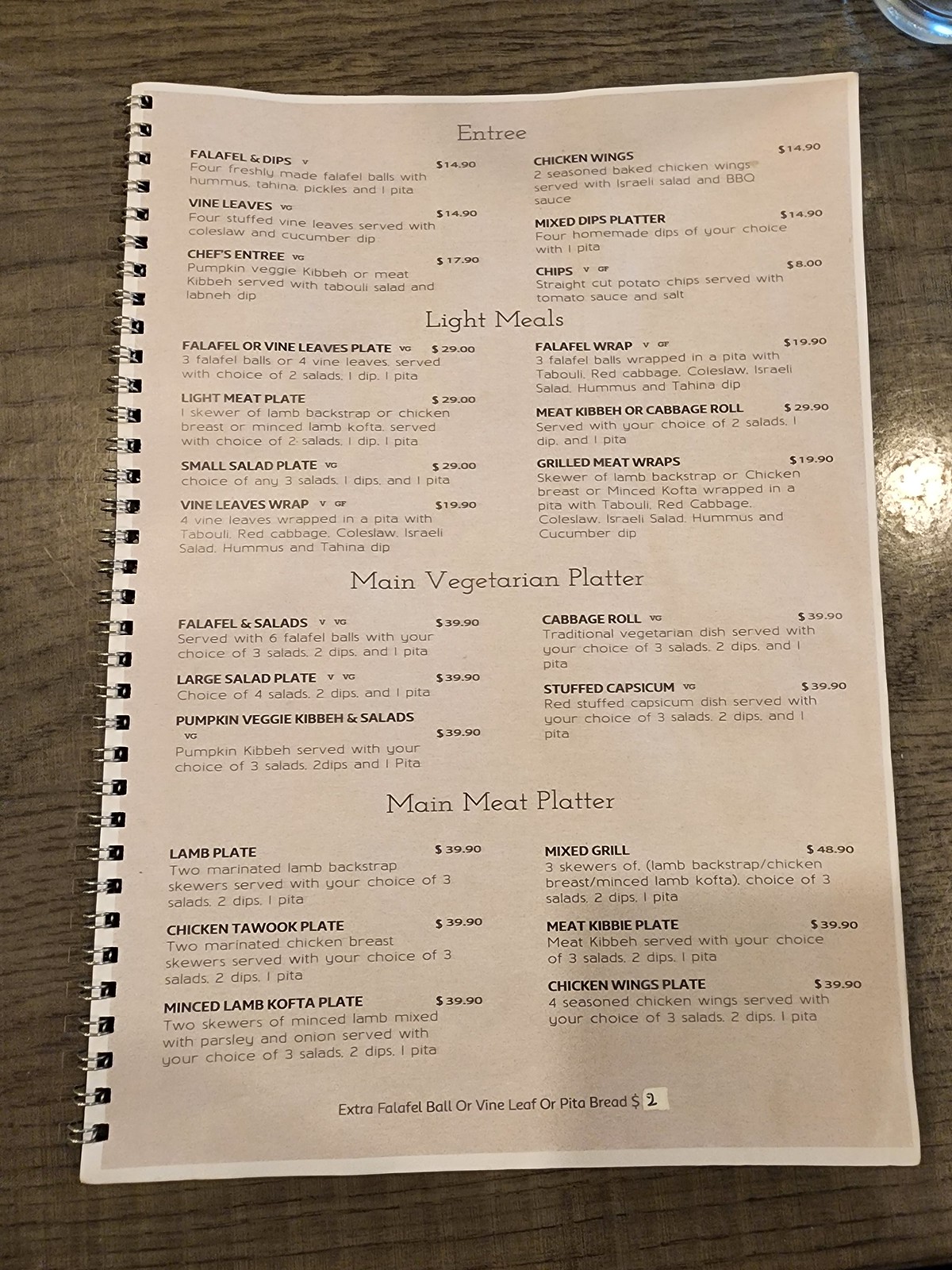This is a clear photo capturing a restaurant menu displayed in a spiral-bound notebook. At the top of the page, the word "Entree" is prominently featured, followed by a list of six entree options. Although the text is slightly out of focus, the visible options include Chef's Entree, Chicken Wings, and Chips. 

Following the entrees, the "Light Meal" section offers a variety of dishes. Despite the readability issue, you can make out offerings such as Vine Leaves Wrap and a small salad plate. 

Further down, the "Vegetarian Platter" section lists five choices, including a large salad plate and a cabbage roll. 

The last section on the page is the "Meat Platter," which features six items, such as mixed grills and a lamb plate.

In the bottom right corner of the image, there is a noticeable shadow in the shape of a square, likely from the smartphone that was used to take the picture. Additionally, there is fine print at the bottom of the menu stating that Extra Pita Bread costs $2.